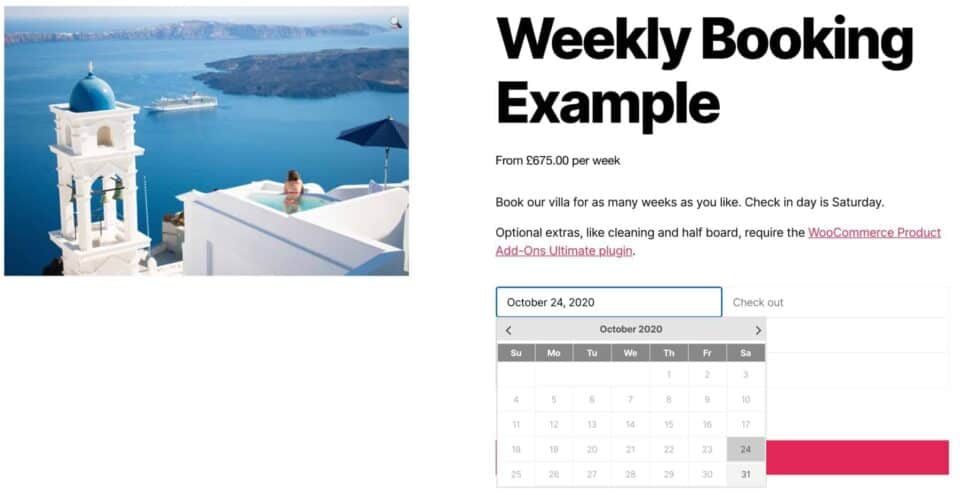**Detailed Caption:**

This screenshot depicts a booking website, evident from the "Weekly Booking Example" header prominently displayed in bold, black text at the top right corner. Below this bold headline, smaller text reads "from £8.75 per week," indicating the cost. Further below, additional details include "Book our villa for as many weeks as you like. Check-in day is Saturday. Optional extras like cleaning and half board require the Web Commerce Product Add-Ons Ultimate Plugin."

The image seems to showcase the villa available for rent—possibly the same one featured at the top left of the screenshot. The villa appears stunning, seen from a high vantage point, potentially from a rooftop relaxation area. The setting boasts a breathtaking view of the ocean, with a large white cruise ship visible in the background, emphasizing the villa's proximity to the sea. Additionally, there is a striking tall white tower on the left side, topped with a baby blue accent, adding to the picturesque charm. The overall aesthetic is characterized by crystal-clear white buildings, enhancing the villa's allure.